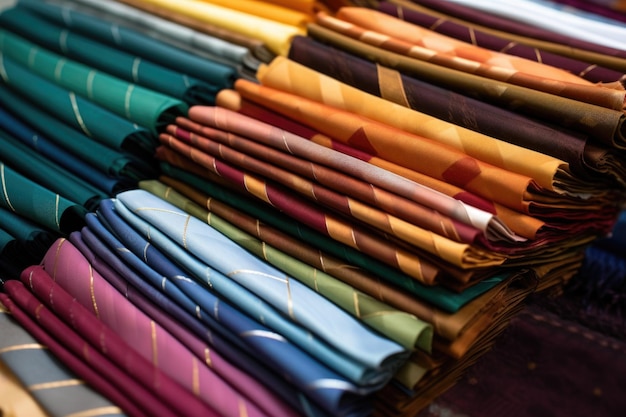The image depicts an intricate arrangement of silk handkerchiefs with a focus on a variety of colors and patterns. The scene features two main stacks of these folded fabrics lying next to each other on a brown background. The central stack starts at the bottom left and stretches to the top right of the frame, showcasing a spectrum of colors that include dark and light pinks, blues, greens, browns, and oranges. Separately, the adjacent stack on the left displays a predominance of turquoise, greenish-blue hues, and hints of gold stripes. Towards the top of this stack, shades transition into yellows and oranges. The bottom right of the image fades into darkness, bringing less visual clarity and minimal hinting at additional stacks. The overall arrangement highlights each vibrant folded piece meticulously layered, creating a textured and colorful display.